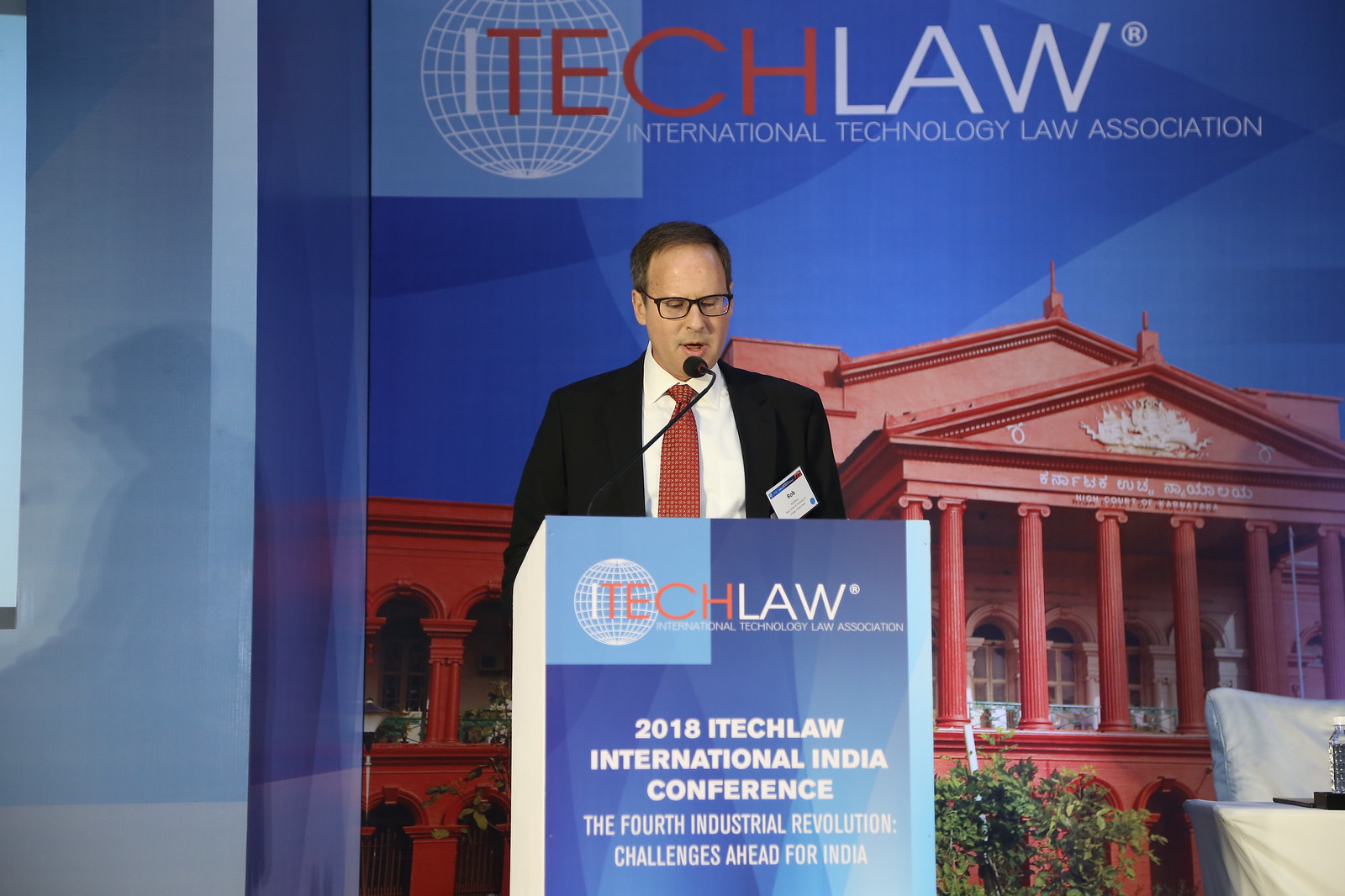The photograph captures a man in a dark suit, white shirt, and red tie standing behind a blue and white podium, addressing an audience at a conference. He’s wearing glasses and has an identification badge displayed on his left chest. The podium prominently features the text "Tech Law, 2018 I-Tech Law International India Conference, The 4th Industrial Revolution: Challenges Ahead for India," in white and orange-red letters. The backdrop behind him includes another banner displaying the same "Tech Law" logo and the title "International Technology Law Association" above an image of a grand, red government-like building with Greek-style columns. To the right of the speaker, there's a table covered with a white tablecloth, holding a bottle of water and a white chair.